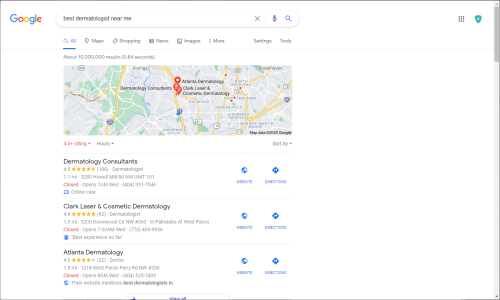The image displays a screenshot of a Google search interface taken from a computer. The background is predominantly white with the iconic Google logo situated in the upper left corner, featuring the familiar colors: blue, red, yellow, blue, green, and red. Central to the image is a search bar containing the query "Best Dermatologist Near Me" written in black text. Adjacent to the search bar, on the right-hand side, are utility icons including an 'X' to close, a microphone symbol, and a magnifying glass representing the search function. Further along the far-right edge, there are three horizontal lines indicating a menu, followed by a shield icon, the purpose of which is unclear.

Directly below the search bar, a navigational menu is highlighted in blue. This menu includes options such as "All" in gray, "Maps," "Shopping," "News," "Images," "More," "Settings," and "Tools," each underlined. Below this, a Google Map is partially visible, shaded in gray, yellow, and green hues, suggesting locations in the Atlanta, Georgia area.

Three dermatology practices listed are "Dermatology Consultants," "Clark Laser and Cosmetic Dermatology," and "Atlanta Dermatology." Beside each listing, there is additional text in light gray, though it is too small and faint to be legible. A scroll bar is present along the right side of the window, positioned at the top. 

In summary, the screenshot captures a detailed Google search result page focused on finding dermatologists near the user, likely located in Atlanta, Georgia.